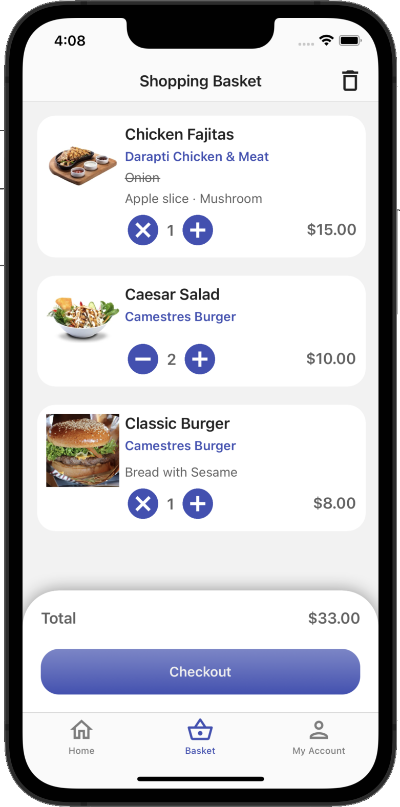A man is depicted using his phone to order food. The phone screen displays the ordering app interface at 4:08 PM, with full Wi-Fi strength and battery life indicators at the top. The screen's header reads "Shopping Basket" in black, accompanied by a trash icon for item deletion on the right.

The ordering interface is divided into three distinct sections, each showcasing a food category with corresponding images and details. The first section features "Chicken Fajitas" prominently displayed in black. Below the title, in blue, it lists "Direppity Chicken and Meat" (spelled D-A-R-A-P-T-I), and notes that onions are excluded, evidenced by an onion symbol with a strikethrough. Additional items include apple slices and mushrooms. The item quantity is adjustable via a blue circle with plus and minus options, currently set to 1 with a price of $15.

The second section displays a picture of a "Caesar Salad" above the title "Masteries Burger" (spelled C-A-M-E-S-T-A-R-E-S burger), currently ordered in a quantity of 2. This item is similarly adjustable but lacks exclusion indicators, priced at $10.

The third section showcases a "Classic Burger" with sesame bread, offering the same add or delete options, priced at $8. 

The cumulative total for the order is $33, with a blue "Checkout" button available beneath the total. At the bottom of the screen, there are navigation icons for Home, Basket, and My Account, with the Basket icon highlighted in blue, indicating the current page.